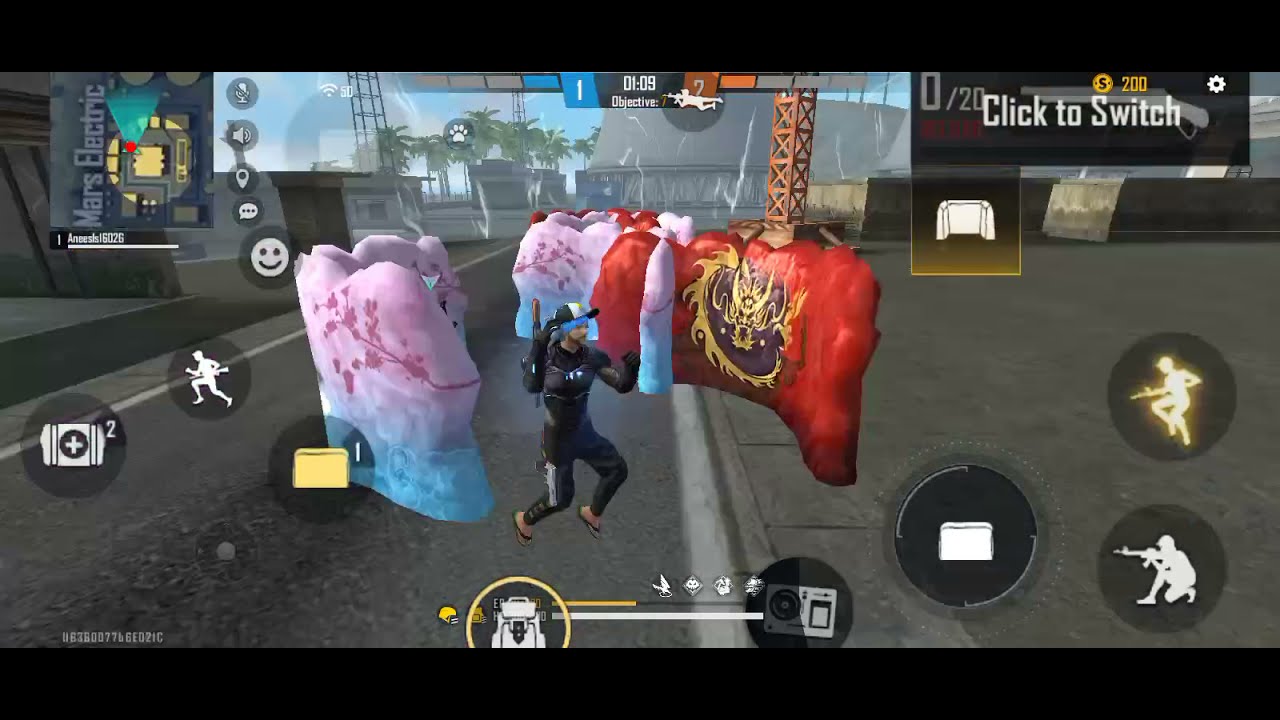In this image, we see a detailed screenshot from an interactive first-person shooter video game set in a dynamic, open cityscape. At the center of the image, slightly off-center to the left, stands a human character. The character has a peach complexion and is equipped with black armor, a white and black hat accented with a blue bandana. This cityscape features vibrant artificial walls in various shades such as pink, blue, red, and yellow, forming protective barriers and structural elements.

The background reveals a sprawling cityscape with industrial elements, such as concrete blocks, pillars, and stands, interspersed with greenery from trees. The sky is a clear blue, suggesting a daytime setting. Various icons and buttons adorn the screen, including a radar in the top left and several interface elements on the bottom and bottom right. Notable text on the screen reads "click to switch objective" and "Mars Electric," likely indicating the map's name.

The image also includes a colorful array of artificial structures with one to the left of the character and another behind him to the right, the latter embellished with a gold and purple dragon crest. The visual style, rich in iconography and vibrant colors, emphasizes the game’s interactive and strategic play, capturing the essence of a fast-paced, immersive video game environment.